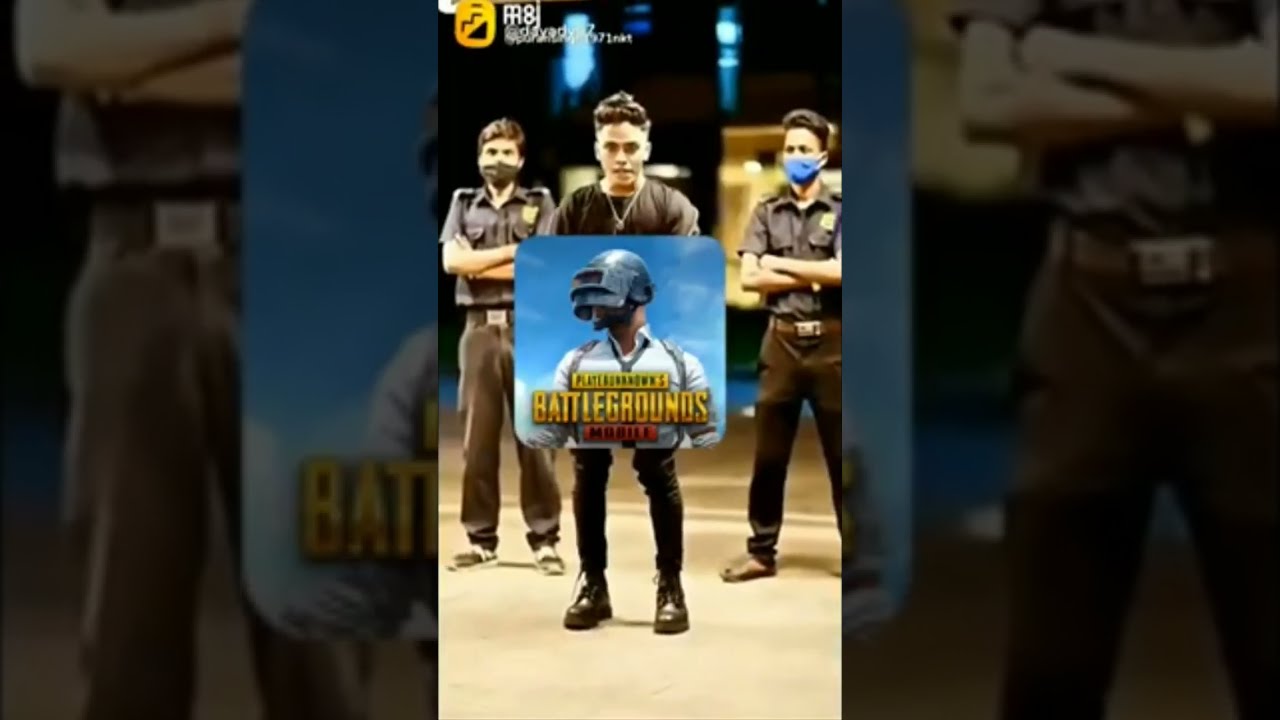This photograph features three men standing in alignment, with the central figure positioned slightly ahead of the other two. The man in the middle, dressed entirely in black with a t-shirt, pants, shoes, and a necklace, is holding a square-shaped billboard. This billboard showcases an image of a man wearing a metal helmet and a white button-down shirt, along with the unmistakable yellow text "Battlegrounds" across his chest, likely referencing the mobile game PlayerUnknown's Battlegrounds.

Flanking behind him are two individuals who appear to be police officers. They both don black shirts and pants, light brown shoes, and belts, and are identifiable by badges on the left side of their shirts. Additionally, both officers have dark black hair, folded arms, and are wearing COVID masks.

The entire scene is superimposed over an enlarged, underexposed version of the same photograph, creating a backdrop effect where the darker, larger background mirrors the central, well-lit image. Surrounding the central image on both sides, this repetition reinforces the emphasis on the main subjects while presenting a layered composition. On top of the central billboard is a logo, and though there are some watermarks and names visible, they appear blurry and overlapping.